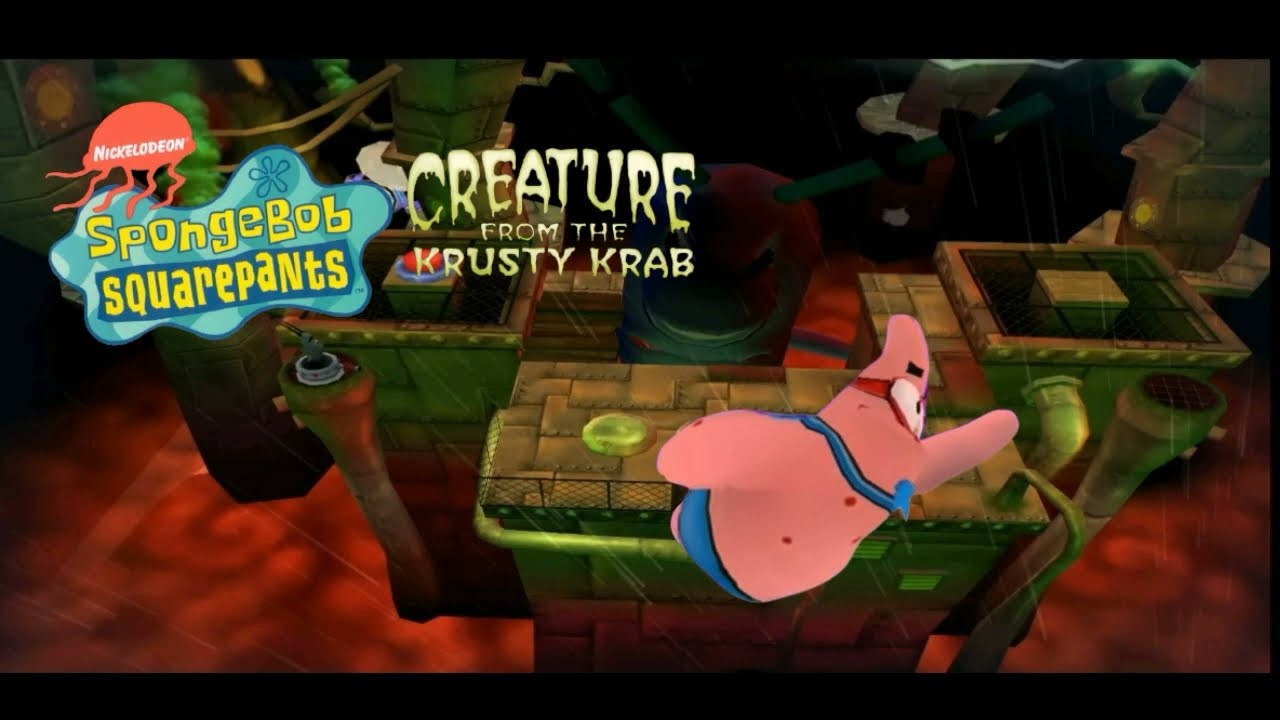The image is an advertisement for a Nickelodeon show, prominently featuring elements from a SpongeBob SquarePants video game, likely titled "Creature from the Krusty Krab." In the upper left corner, there's an orange-colored, octopus-shaped cartoon figure with the word "Nickelodeon" in white lettering. Directly below this is a blue liquid splotch with "SpongeBob SquarePants" written in yellow on it. Positioned to the right, the title "Creature from the Krusty Krab" is displayed in yellowish-white text.

The focal point of the image is a pink, starfish-like character, likely Patrick, who is adorned with blue shorts, a blue strap around his belly, and red goggles with white lenses held by a red strap around his head. He also appears to be wearing a cape-like blue strap around his neck. Patrick has one arm extended forward without a visible hand and another arm reaching backward. The background features an arrangement of variously shaped tiles, creating a visually engaging, puzzle-like effect. There are stone walls and metal pipes, suggesting an obstacle course setting. At the bottom of the image, it looks like there's a pool of lava, adding a sense of danger or excitement, with Patrick seemingly floating above the platform.